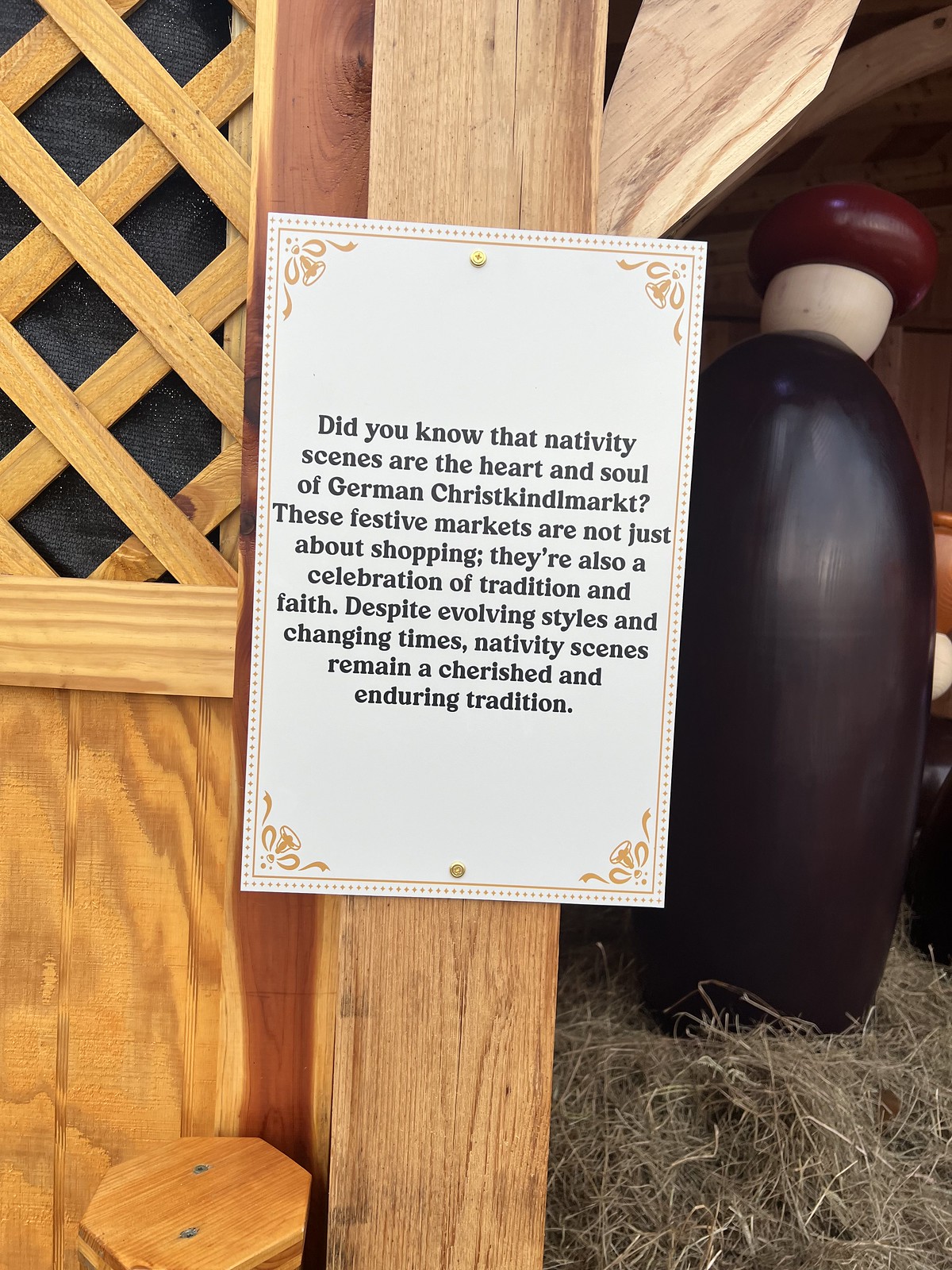A detailed sign is affixed to the top and bottom of a light-colored wooden post, set against a backdrop of wood lattice work and boards. The sign, adorned with a decorative outline featuring inward-reaching golden bells and ribbons at each corner, reads: "Did you know that nativity scenes are the heart and soul of German Christkindl markets? These festive markets are not just about shopping. They're also a celebration of tradition and faith. Despite evolving styles and changing times, nativity scenes remain a cherished and enduring tradition." To the left of the sign, there is more visible wood lattice work, while to the right, partially obstructed by hay, is a simplistic wooden human figure consisting of an oblong body and featureless head, wearing a red wooden turban. The scene suggests a festive and traditional display central to the German Christkindl market experience.